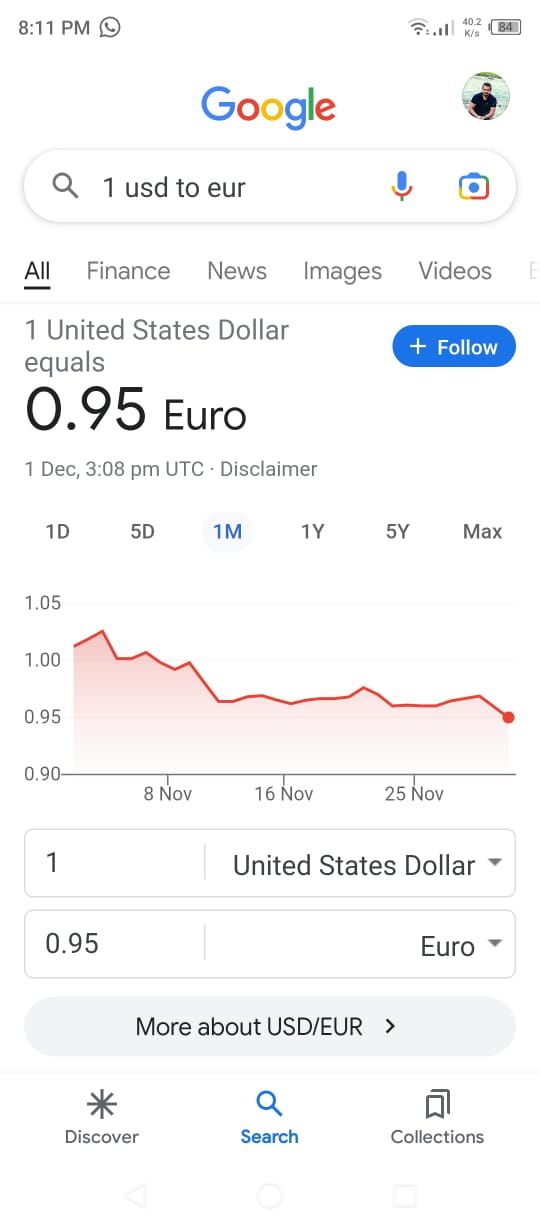Screenshot description:

This screenshot from a cell phone displays a white background. 

**Top Information Bar:**
- **Top left corner:** "8-11pm"
- **Top right corner indicators:**
  - **WiFi signal:** 3 out of 4 bars
  - **Carrier signal:** 3 out of 4 bars
  - **Data speed:** 40.2 kilobytes per second
  - **Battery level:** 84%

**Google Search Interface:**
- **Google Logo:** Displayed in its classic blue, red, yellow, and green letters
- **Profile Picture:** To the right of the logo, there is an image of a man seated in front of what appears to be a river.

**Search Bar:**
- Shows the query: "1 USD to EUR"
- **Microphone and camera icons:** Present on the right side of the search bar

**Search Options:** 
- **Tabs below the search bar:** "All" (selected), "Finance", "News", "Images", and "Videos"
- **Grey underline:** Divides the options

**Search Result Panel:**
- Shows: "1 USD equals 0.95 EUR"
- **Action Button:** To the right, there is a blue oval button with a plus sign and the word "Follow".

**Currency Graph:**
- **Timeframe Options:** "1D", "5D", "1M" (selected with blue highlight and grey circle around it), "1Y", "5Y", and "Max"
- **Graph Axes:**
  - **Y-axis labels:** 1.05, 1.00, 0.95, 0.90
  - **X-axis labels:** 8N, 8N, 16N, 25N
- **Graph Line:** Red with varying shades of pink beneath it; starts just above 1, fluctuates, peaks, and declines to 0.95 with a red dot at the end.

**Conversion Inputs:**
- **Row 1:**
  - **Left box:** "1" in bold, "United States Dollar" with a drop-down arrow
  - **Right box:** "0.95" and "Euro" with a drop-down arrow
- **Action Button:** Grey oval stating, "more about USD / EUR" followed by a right arrow

**Footer Navigation:**
- **Selected Icon:** "Search" with a blue highlight and a magnifying glass icon above it
- **Other Icons:** "Discover" with a star icon, "Collections" with a bookmark icon

**Bottom Navigation Bar:**
- Includes light grey icons:
  - **Triangle**
  - **Circle**
  - **Square**

This comprehensive depiction provides a detailed account of the key features and layout present in the cell phone screenshot.